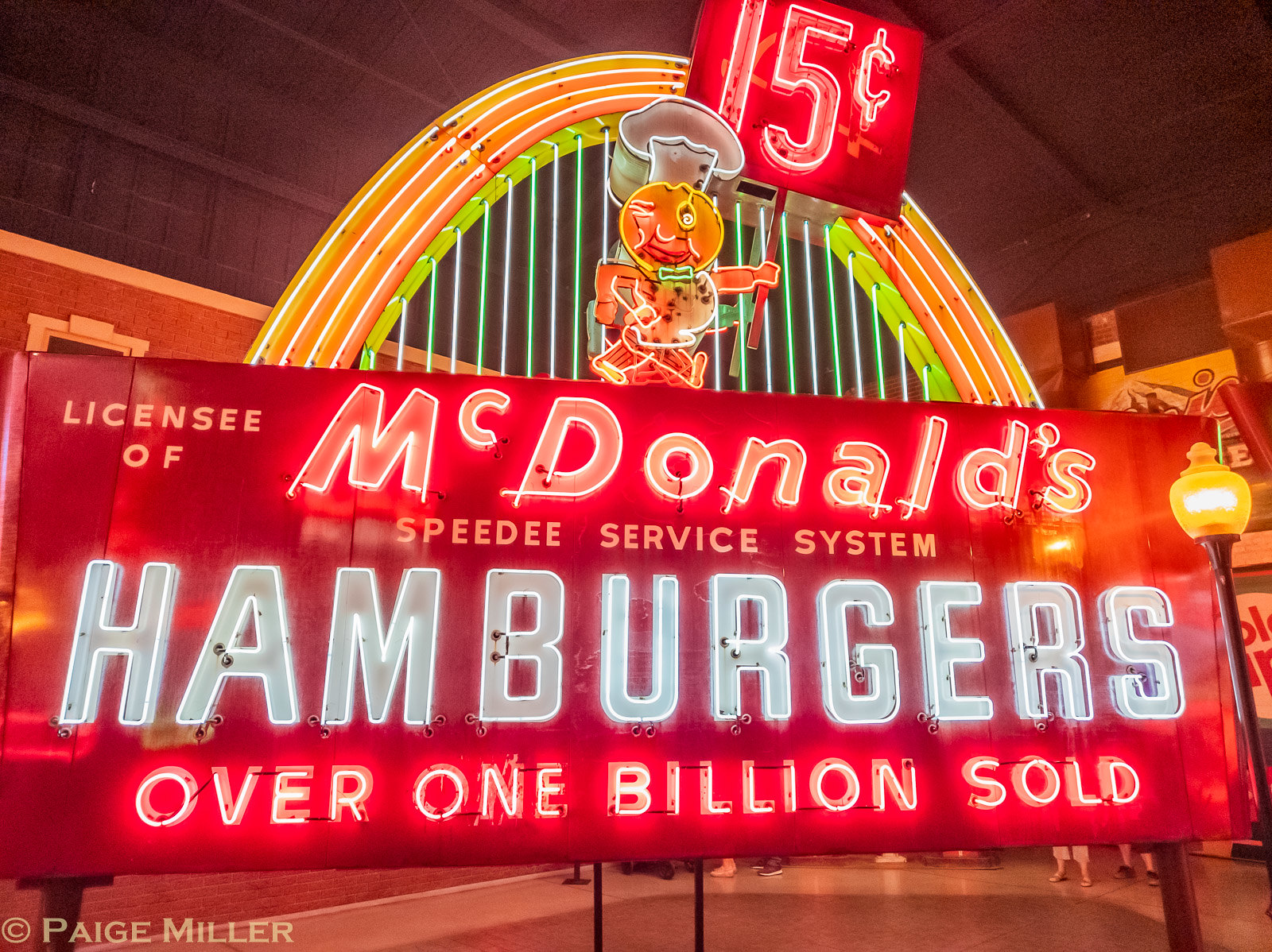This professional photograph captures a vintage, illuminated McDonald's sign, evocative of the chain's early days. The red rectangular sign is centrally lit with bold white neon lettering that reads, "Licensee of McDonald's," followed by "SPEEDY SERVICE SYSTEM," "HAMBURGERS," and "OVER 1 BILLION SOLD." Above this primary sign, a vibrant arch composed of yellow, lime green, and orange neon bulbs loops over it, reinforced by many illuminated posts. At the pinnacle of the arch, a distinctive neon figure stands out: a stylized hamburger donning a white chef's hat, with leg-like elements suggesting movement, but it's clearly stationary. The figure holds a smaller red sign proclaiming "15 cents" in bright white numbers. This sign isn't affixed to a building; instead, it seems freestanding, possibly located indoors as indicated by the visible ceiling and floor, which are brown and off-white, respectively. Adding to the image's authenticity and standing, the bottom left corner features a copyright mark reading "PAIGE MILLER." Beneath the sign, partially visible are the feet and shins of people, hinting that this photograph was taken in a populated setting, likely at night given the sign's illumination and the surrounding darkness.